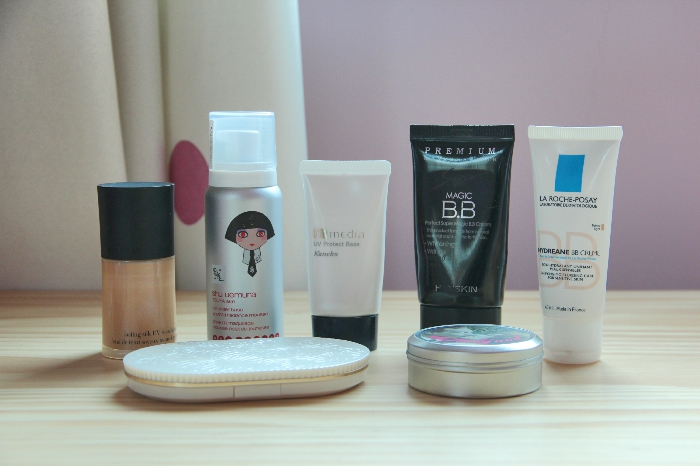A cozy, personal space is depicted in this image, featuring a mauve-colored wall situated on the right-hand side. Adjacent to this wall, on the left, are partially visible cream-colored curtains that add a touch of elegance to the setting. Dominating the foreground is a wood-look countertop or table, which appears to be crafted from a material mimicking wood rather than genuine timber.

Neatly arranged on this countertop are various personal grooming items, creating an organized display. Firstly, there's a bottle of foundation with a black cap, characterized by its round shape; however, the brand name remains illegible. Beside it, a silver bottle, likely containing hair mousse, stands out with its intricate design featuring an illustration of a woman with a bowl cut, red eyes, and a tie.

Following this is a small tube, indistinctly labeled, that suggests a skincare product such as face lotion or an extra firming cream. Another notable item is a tube of 'BB Magic,' encased in a black container with prominent silver lettering, the specific purpose of which remains uncertain. Lastly, a compact lies at the forefront of the arrangement, completing the assortment of personal care items on display.